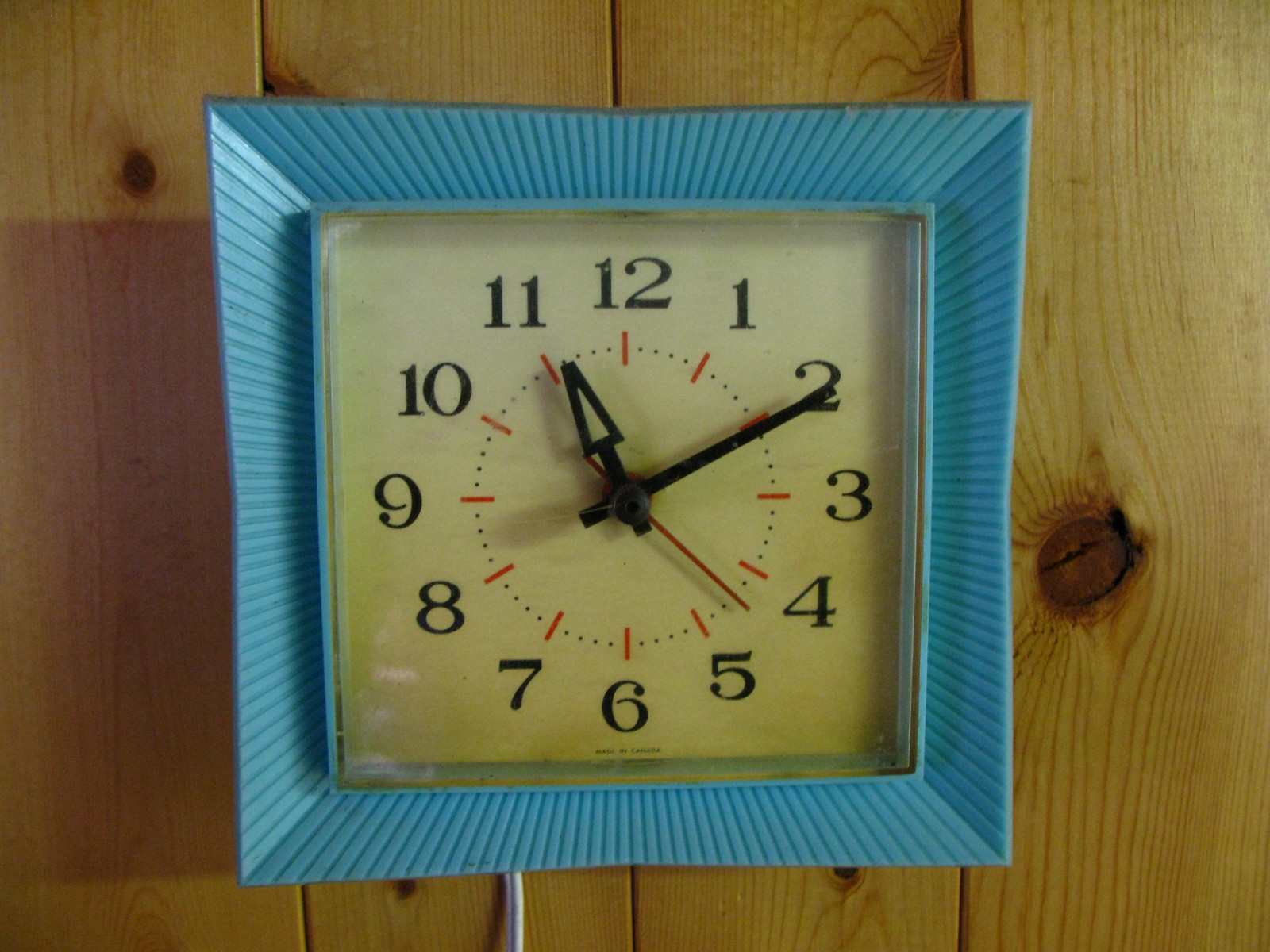This image captures a square wall clock with a box-like appearance. The clock features Arabic numerals from 1 to 12 and includes three hands: an hour hand, a minute hand, and a second hand. The time displayed is approximately 11:11. The photograph is taken during the daytime, as indicated by the natural sunlight illuminating the scene.